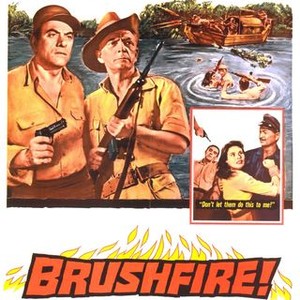This illustrated advertisement for the show "BRUSHFIRE!" features a dynamic scene embodying a 1950s aesthetic. Dominating the composition are two middle-aged men, both armed; one is wielding an AK-47-style rifle while wearing a safari hat, and the other holds a handgun and sports a baseball cap, with both clad in khaki shirts. They're depicted in a tense stance, gazing into the distance, suggesting imminent action. Above them, a tumultuous scene unfolds involving a sinking boat, crocodiles, and people—including a woman, likely being rescued—engaged in a chaotic struggle in the river. Another inset scene shows a woman being restrained by a police officer, with tension evident as a man points a gun at another unseen person in the background. The title "BRUSHFIRE!" is emblazoned at the bottom in bold, orange letters highlighted in black, with dramatic flames behind it, amplifying the excitement and urgency of the show.